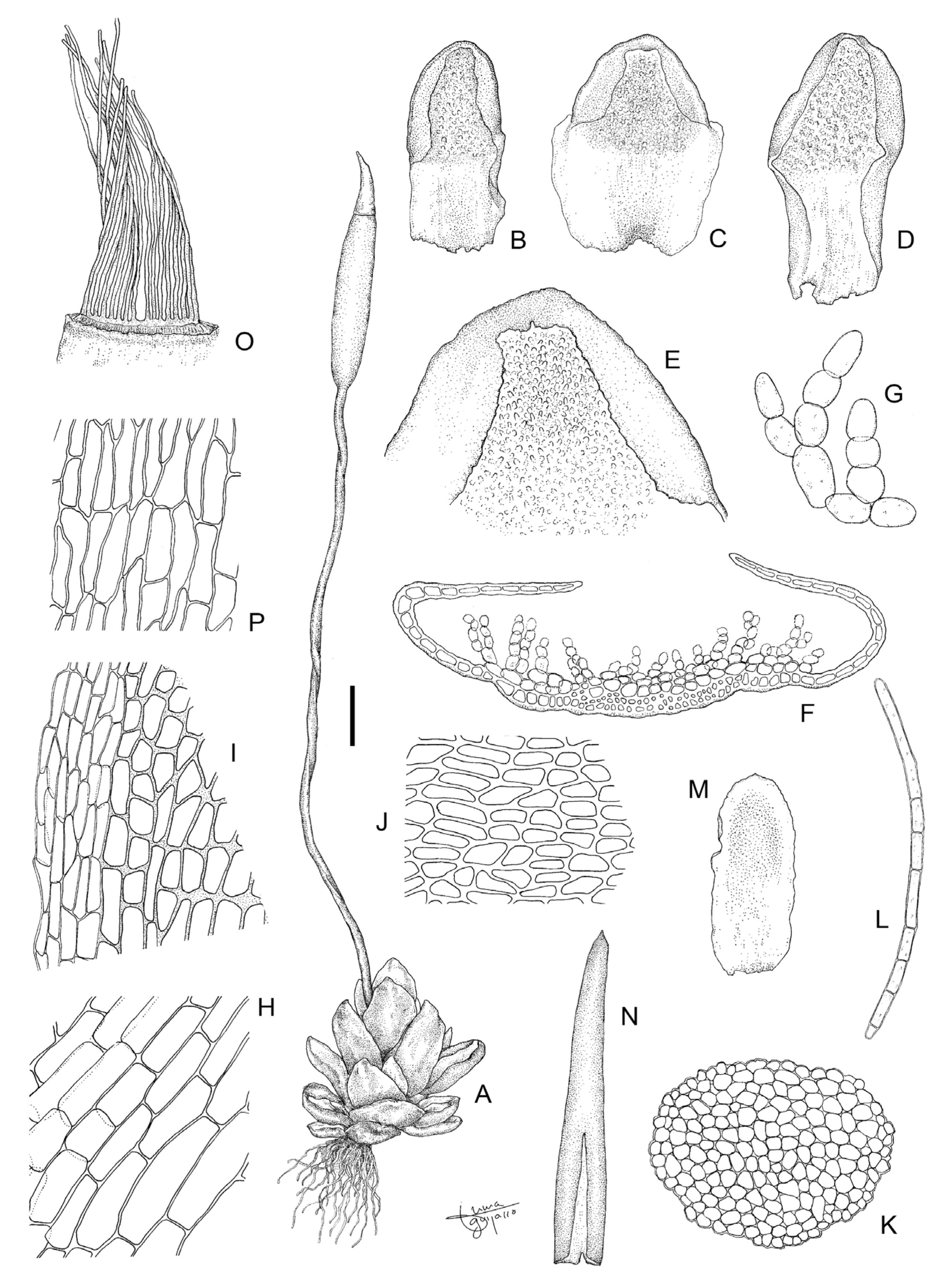This black-and-white infographic presents a detailed array of plant part sketches and diagrams, each labeled with letters from A through P. The illustrations vary in style and complexity, ranging from a flower with a long stem to potential microscopic views of plant cells. These cells are depicted in a variety of shapes, some resembling rows and columns of circles or rectangles, while others mimic irregular stones or blobs. On the lower left-hand side, the letter H marks a drawing of rectangles arranged in a cobblestone or brick pattern. Above this, similar patterns with varying widths and lengths are marked with I and P. Each figure throughout the image is meticulously labeled, and the letters provide a sequence to follow, showcasing different structural aspects of the plant, from roots to buds. The entire composition, seemingly rendered in pencil, emphasizes scientific observation and detailed study of plant morphology.